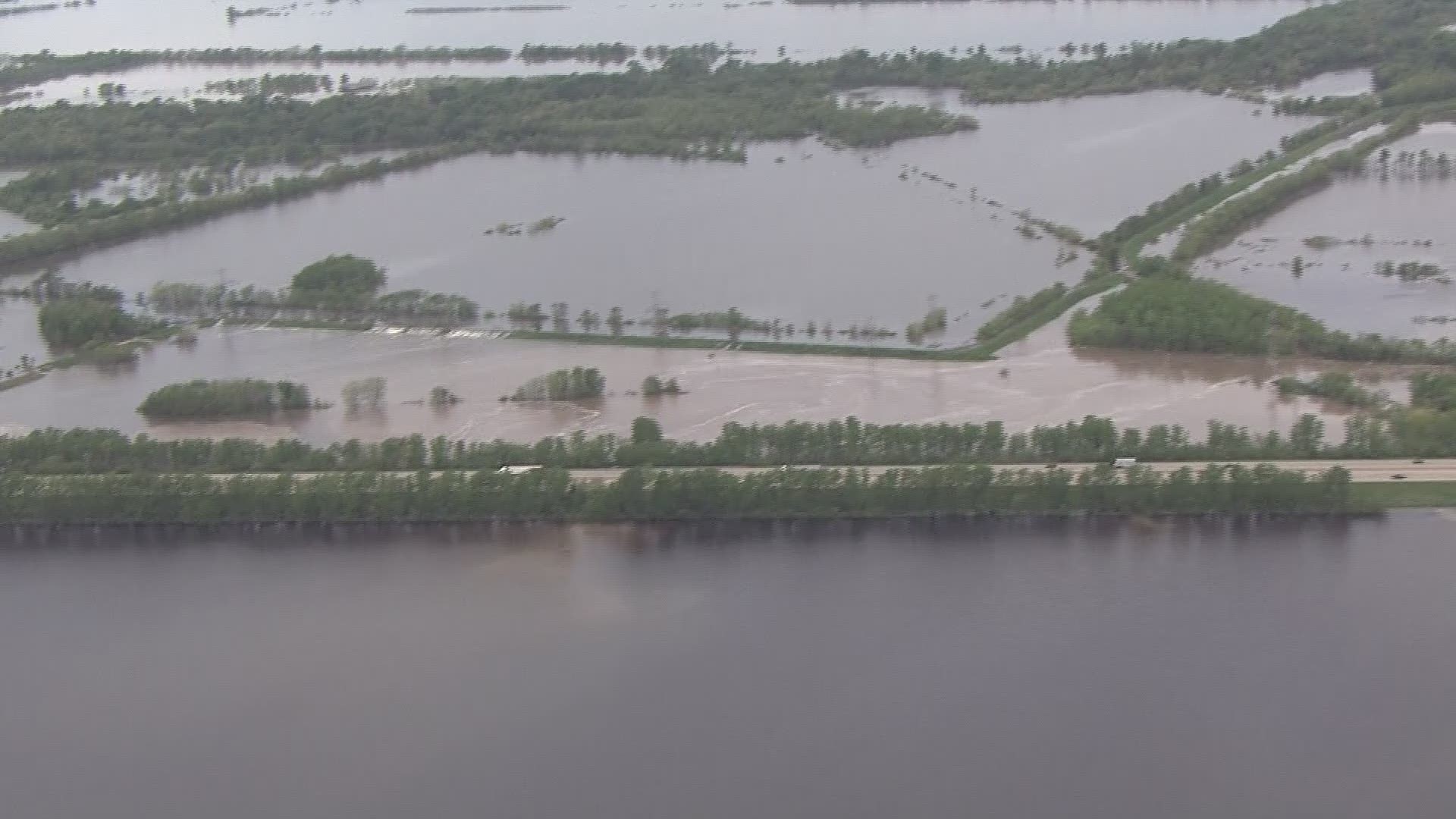This is an aerial view of a landscape featuring a significant presence of both water and land, suggestive of flooding in certain areas. Dominating the center of the image is a four-lane road, slightly elevated, with cars traveling in both directions. This road stretches from the middle left to the middle right of the frame. Below the road, a substantial body of water extends across the entire width of the image, indicating potential flooding. Above the road, a dense line of trees runs parallel to it, also stretching from left to right. Beyond the trees, water continues to be prevalent, interspersed with more trees, suggesting an ongoing flooded region. On the right center of the image, an area with brown water can be seen, bordered by another line of trees that curves slightly downward and then upward to the right. A channel of water navigates through these trees, adding to the overall watery landscape. On the left side of the image, particularly towards the top, sits a dense wooded area. Below this wooded section and to the left, green patches dot the water, presenting a mix of vegetated and submerged land. Along the top of the image, the landscape transitions into more green areas with some water, culminating in a verdant region at the top right-hand corner. Overall, the image is a blend of flooded lands, interspersed with roads, trees, and occasional green patches, painting a detailed picture of a water-rich environment.